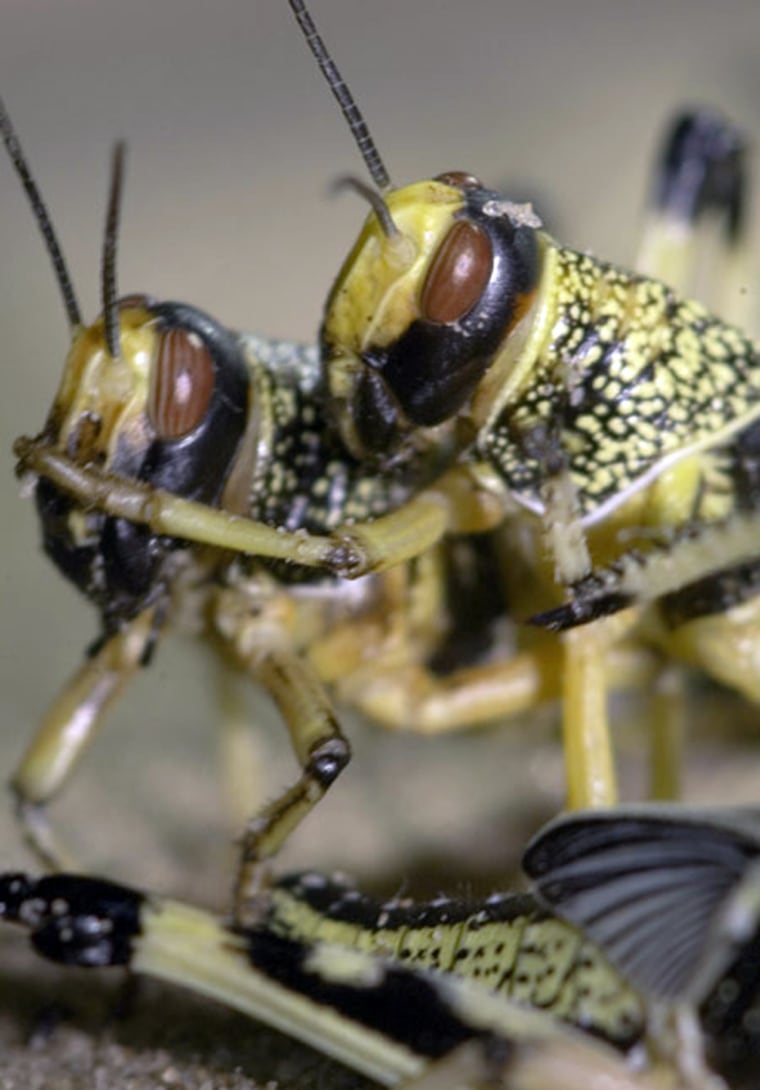The image captures two insects that appear to be interacting closely with each other. These winged insects exhibit a striking coloration of yellow and black markings. Both insects have almond-shaped brown eyes, surrounded by white accents. Their antennae are distinctly black. The bodies of the insects feature a yellow base with black spots, and the legs are a yellowish-green color with black markings. One insect seems to be gently touching the other with its leg, giving the appearance of an embrace. They are standing on a brown, dirt-like surface. The background is blurred, drawing focus to the insects. There is a hint of another insect in the bottom right corner, mostly cropped out of the image. While their exact species is unclear, they resemble bees, moths, crickets, or even grasshoppers.